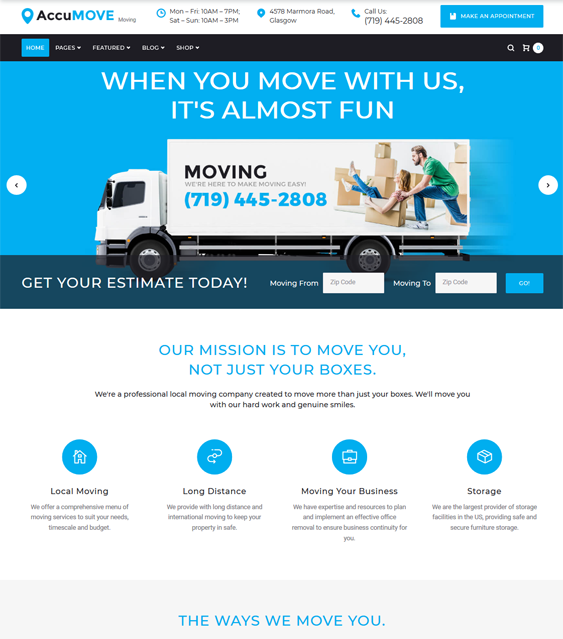This is a detailed description of a web page belonging to a business called AccuMove:

---

**Website Overview for AccuMove:**

**AccuMove (A-C-C-U M-O-V-E) Business Website**

- **Visual Icons and Text on the Left Side:**
  - **Pinpoint Icon:** Accompanied by the word "moving."
  - **Clock Icon:** Indicates operating hours:
    - **Weekdays (Monday through Friday):** 10 a.m. to 7 p.m.
    - **Weekends (Saturday and Sunday):** 10 a.m. to 3 p.m.
  - **Pinpoint Icon:** Displays the address "34578 Marmora Road, Glasgow."
  - **Call Us:** Specified phone number "719-445-2808" noted in parentheses.

**Top Right Section:**
- **Appointment Button:** Rectangular button with "Make an Appointment" in white text alongside a dog icon.

**Navigation Banner:**
- **Menu Items in White Text on a Black Banner:**
  - Home
  - Pages
  - Featured Blog
  - Shop
  - Right side: Search icon, car icon, and an unidentified icon.

**Central Main Section:**
- **Background:** Blue.
- **White Moving Truck:** Featuring the text "Moving."
- **Promotional Text:** "We're here to make moving easy," along with their phone number.
- **Imagery:** Picture of two people holding boxes.
- **Text Above Image:** "When you move with us it’s almost fun."

**Bottom Section:**
- **Estimate Request:**
  - **Icon:** Dark blue.
  - **Text:** 
    - "Get your estimate today."
    - "Moving from" (with a box for zip code).
    - "Moving to" (with a box for zip code).
  - **Action Button:** "Go."
- **Mission Statement:** 
  - "Our mission is to move you, not just your boxes."
  - "We’re a professional local moving company created to move more than just your boxes. We’ll move you with our hard work and genuine smiles."

**Service Icons (Four Blue Round Icons with White Graphics):**
  - **Home Icon:** Local Moving - "We offer a comprehensive menu of moving services to suit your needs, timescale, and budget."
  - **Arrow Icon:** Long Distance - "We provide long distance and international moving to keep your property safe."
  - **Building Icon:** Moving Your Business - "We have the expertise and resources to plan and implement an effective office removal to ensure business continuity for you."
  - **Storage Icon:** Storage - "We’re the largest provider of storage facilities in the U.S., providing safe and secure furniture storage."

**Footer:**
- **Light Gray Banner:** "The ways we move you" in blue text.

---

This descriptive caption gives a comprehensive overview of the AccuMove business website, detailing its layout, features, and key elements.